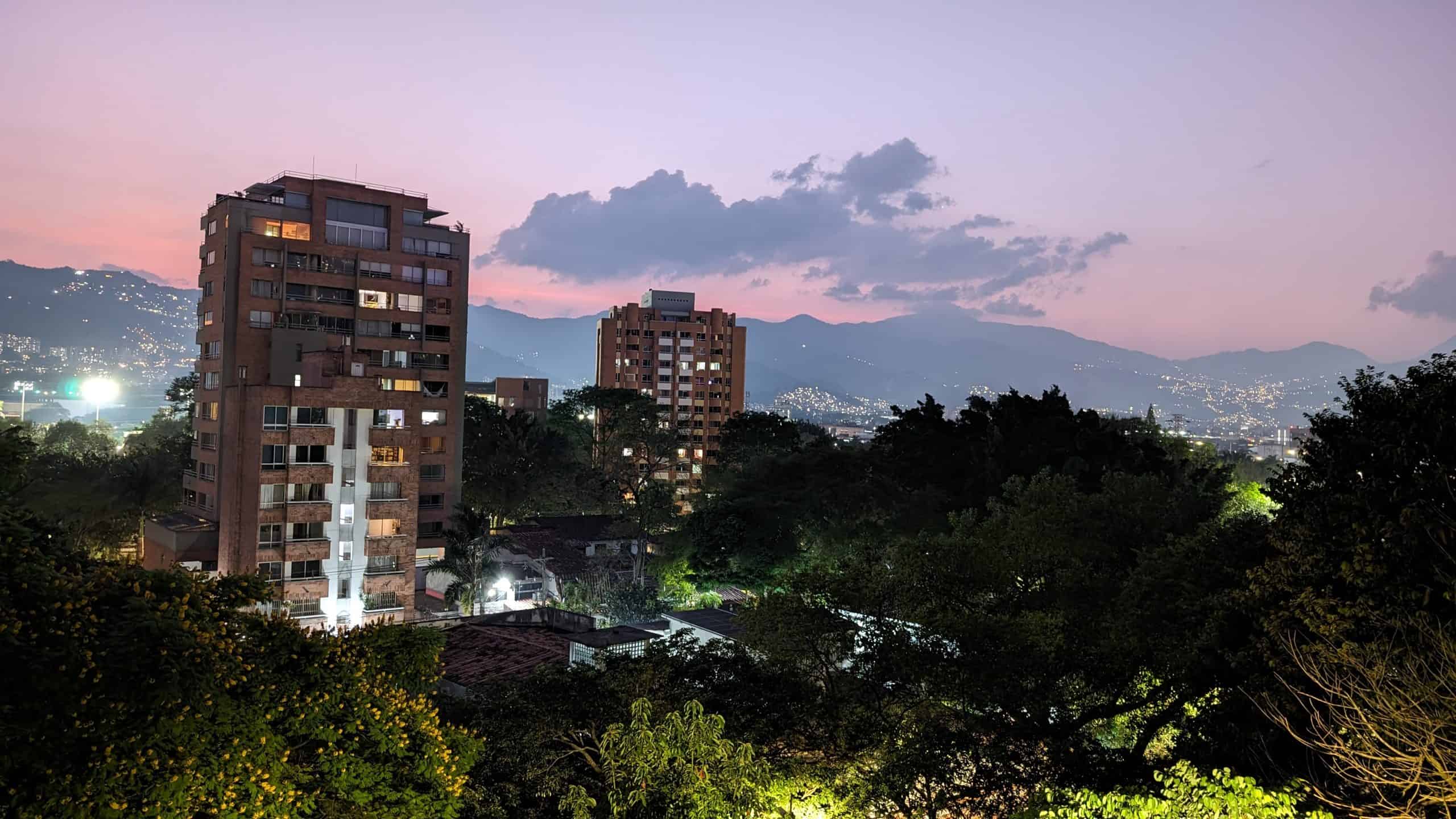This aerial photograph, taken at dusk, features two tall, red brick high-rise apartment buildings, each standing over 10 stories tall. The closer building is positioned on the left, while the other stands slightly further back and to the center. They overlook a lush, green area abundant with tall trees and scattered shrubs, suggesting a heavily wooded residential neighborhood. Streetlights cast an inviting glow over the trees in the foreground, hinting at a well-maintained area. To the rear of the buildings, nestled in a lower-lying area, one can glimpse a pool and possibly other residential houses. The scene extends to a distant valley peppered with city lights, marking the presence of streets and additional buildings obscured in shadows. Beyond this, a serene mountain range forms a dramatic backdrop under a soft orange and purple sunset, with a mostly clear sky dotted by a few wispy clouds. The overall impression is that of a tranquil, elevated residential area within close proximity to a bustling city, captured beautifully during the twilight hour.